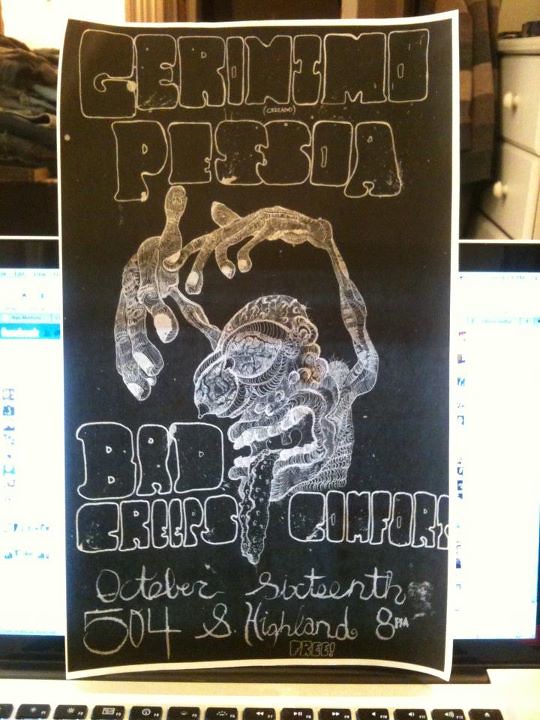The image is of a black sign with a white border, featuring a heavily stylized cartoon caricature centered on a piece of white paper printed with black ink. At the top, thick, chunky, rounded text reads "Geronimo Pessoa." Below is a striking illustration of a malnourished creature with a disproportionately large head, bugging eyes that jut from its sockets, and a gaping mouth with a tongue hanging out. The figure's thin, elongated arms have enormous hands that arch above its head, further emphasizing its exaggerated features. Beneath the illustration, additional text reads "bad creeps comfort." Smaller text at the bottom details event information: "October 16th, 5048 Highland, 8 pm free." The sign rests in front of a laptop screen, hinting at a living room or bedroom setting in the background. This surreal and grotesque visual primarily serves as an ad for a college party event.